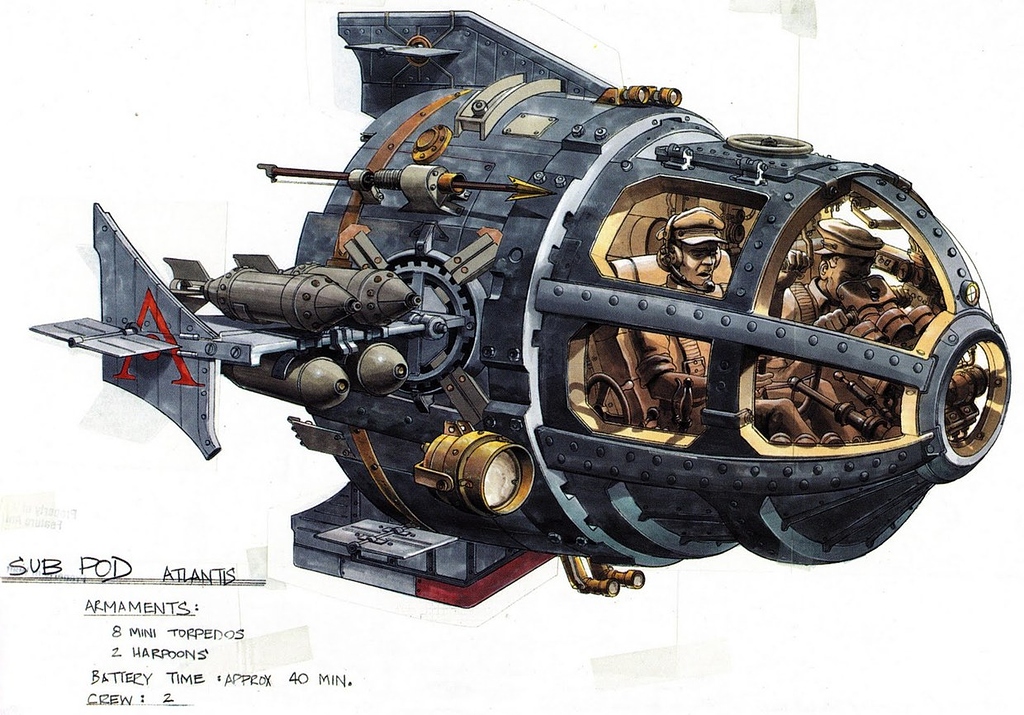The image is a colored pencil illustration of a military underwater craft named "Subpod Atlantis." The vehicle, primarily gray with gold embellishments, has a robust tubular structure that combines features of both a submarine and a spacecraft, including metallic wings adorned with at least four missiles. Prominently displayed on one fin is a red letter "A". The front section of the craft is translucent, forming a steel-reinforced cockpit with metal bars and windows, allowing for extensive underwater observation. Inside the cockpit are two army-clad men, each wearing headsets and hats, with wristbands situated just above their elbows. The man at the front is peering through a binocular-like device. A harpoon shooter is mounted on the top left, and additional equipment includes a large lamp and scope on the fuselage, alongside a door hatch. Detailed text on the bottom left of the drawing specifies: "Subpod Atlantis, armaments: eight mini torpedoes, two harpoons, battery time approximately 40 minutes, crew: two." The interior lining and certain ocular features also exhibit a gold finish.